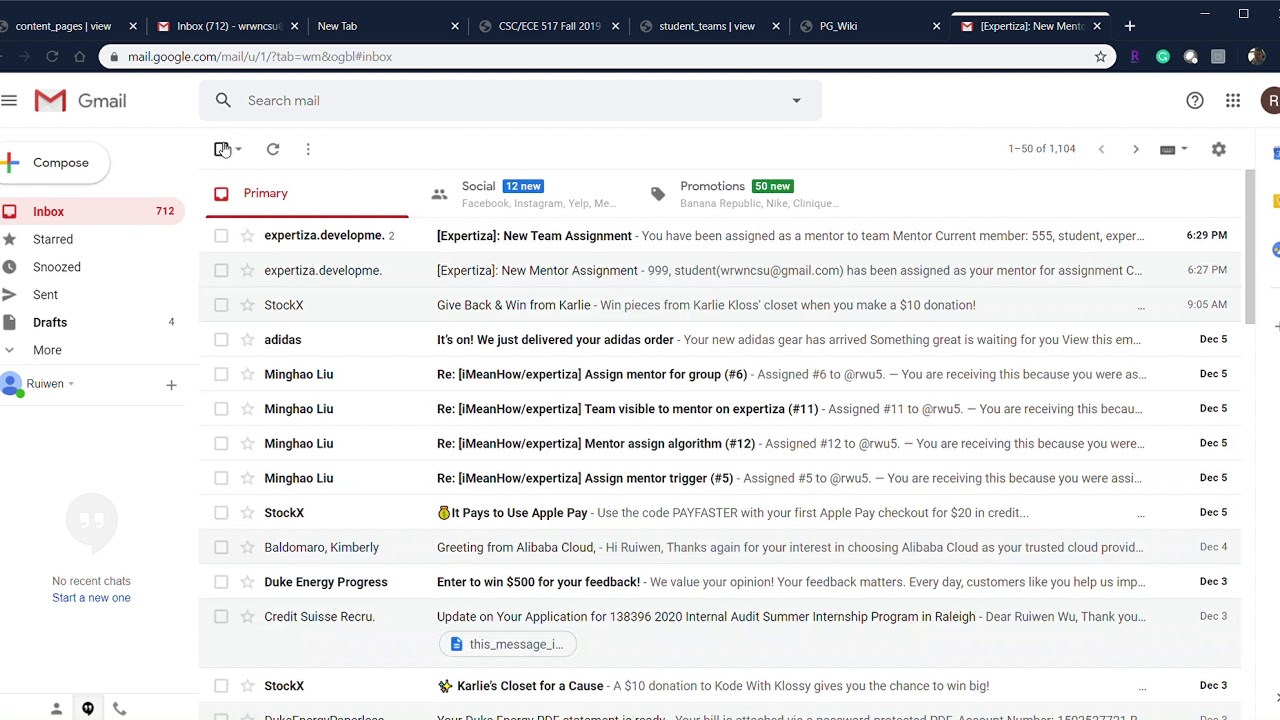This screenshot shows a computer browser with seven tabs open, with the seventh tab selected on the far right of the browser window. The active tab is displaying the Gmail interface, as indicated by the URL "mail.google.com" in the search bar beneath the tabs. On the left side of the interface, there is a navigation menu featuring options such as Inbox, Starred, Snoozed, Sent, Drafts, and more, which can be expanded using a toggle switch. The central area of the screenshot reveals a list of approximately 10 to 15 emails. Many of these emails appear unread, denoted by bold black text, while others are read and displayed in a thinner, gray text. The dates of the emails are shown in the right-hand column.